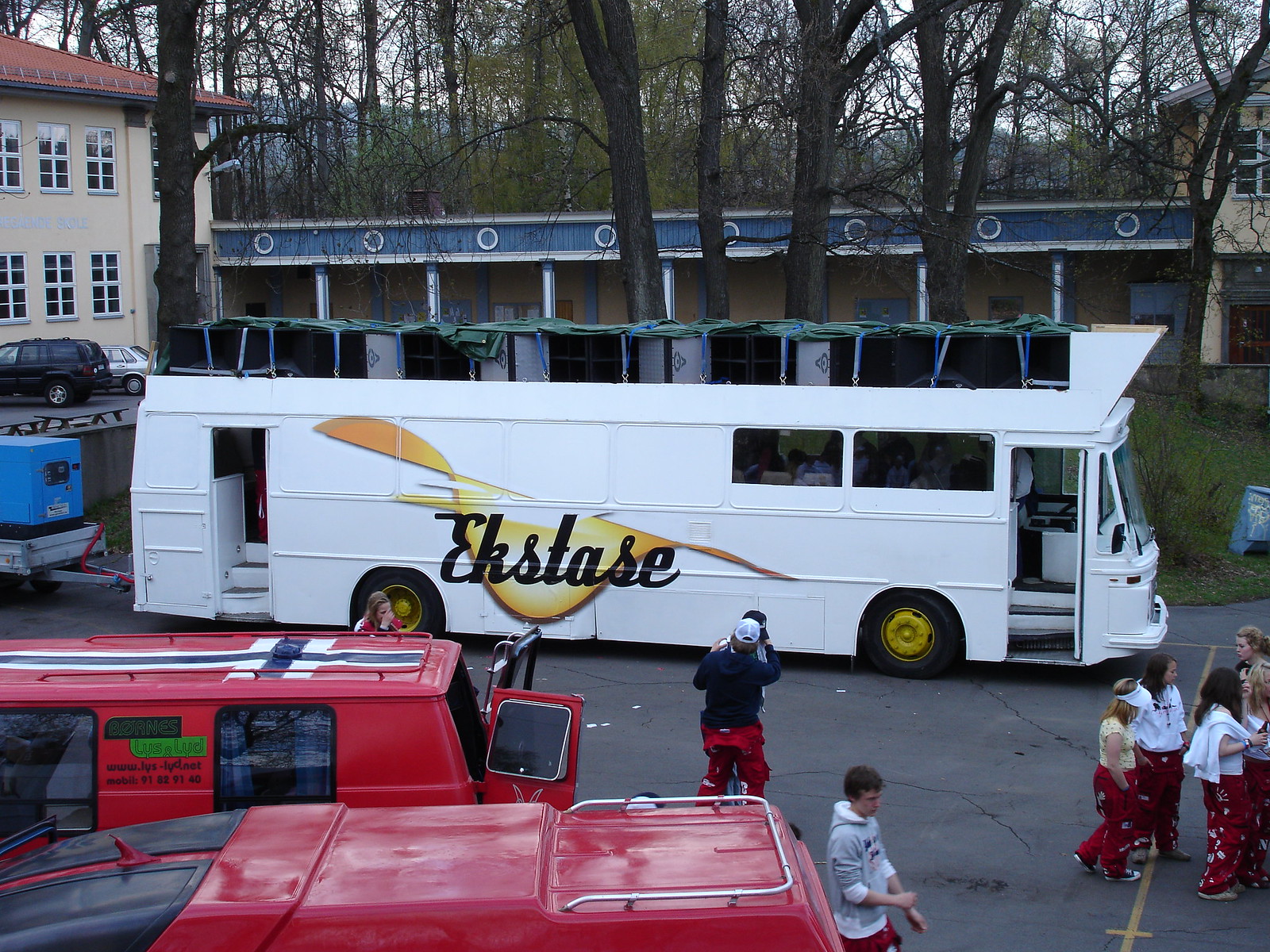The image showcases a busy street scene with a prominent white charter bus at its center. The bus, with black tires and distinctive yellow rims, has the word "E-K-S-T-A-S-E" emblazoned in black cursive lettering along its side. The bus features both a front and a rear entry door, each with windows. On top, various black storage cases, possibly speakers, are secured and partially covered by green tarps.

In the foreground, several vehicles, including multiple red vans, are visible. The rear doors of one such van are open, revealing an interior view. One van's roof is painted with the Finnish flag. A number of people are seen milling around, with some standing and others on bicycles. A notable figure is a man in red pants, a blue shirt, and a white hat, who appears to be consoling another man wearing a hat. Nearby, a woman sits beside one of the red vans, which bears green lettering.

Several women, uniform in red pants and mostly white shirts, with one wearing a yellow shirt and visor, stand near the bus. The street is marked by a yellow line, and in the background, a two-story residential building and various trees, possibly part of a park, add depth to the scene.